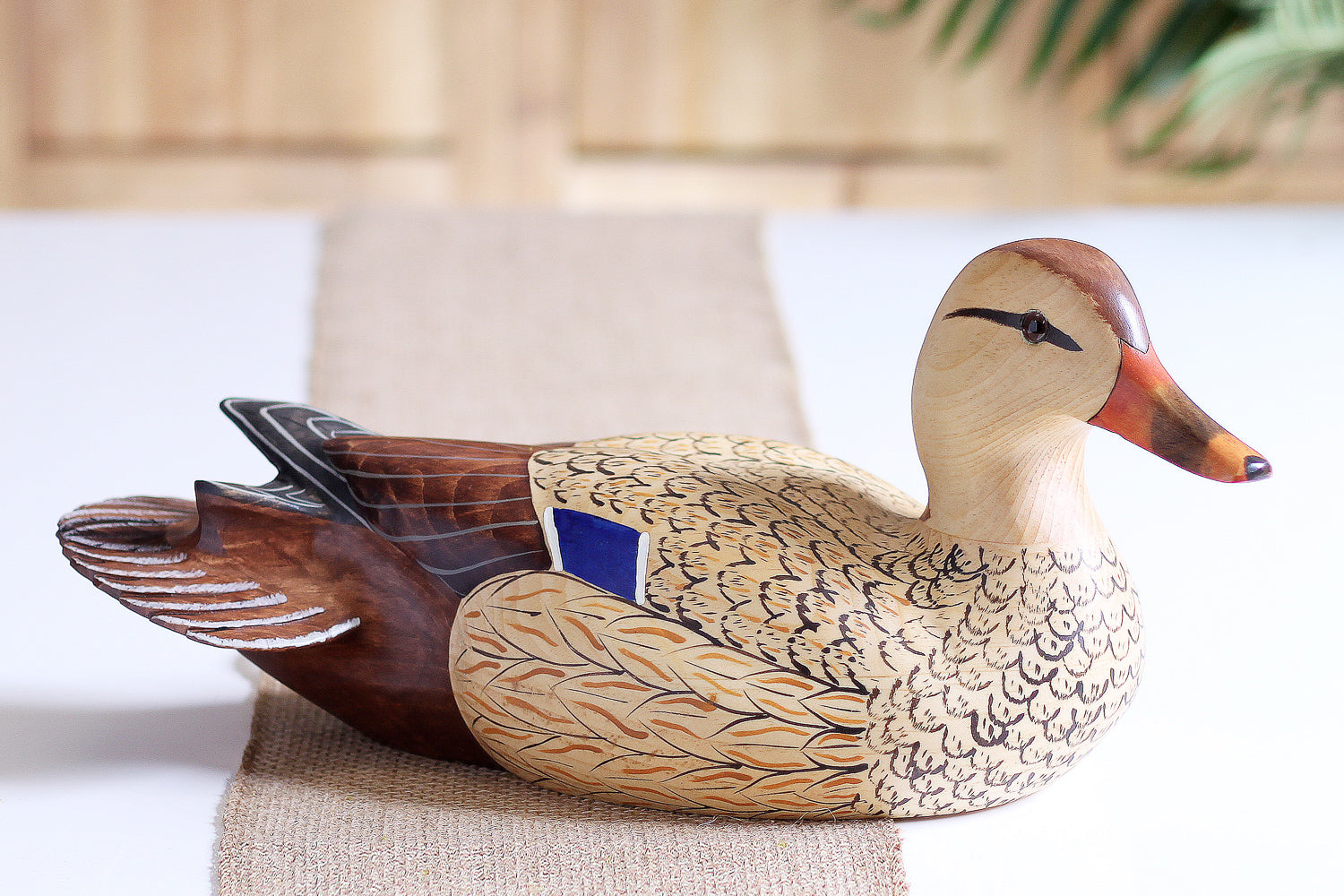This photograph captures a detailed scene of a wooden mallard duck decoy placed on a white countertop. The countertop features a burlap-style table runner that extends from the background to the foreground. The decoy is crafted with a cream-colored head and body, adorned with a dark brown back and tail feathers. A distinctive blue square is located in the middle of what would be the wing area. The duck's beak showcases shades of orange and brown, with a black stripe running across and down its head to the beak. The eye is marked with a black line. In the background, slightly out of focus, are wood-grained cabinets, with a green plant visible in the top right corner. The lighting, coming from the right-hand side of the photograph, casts a shadow that enhances the three-dimensionality of the decoy, which is facing to the right of the image.